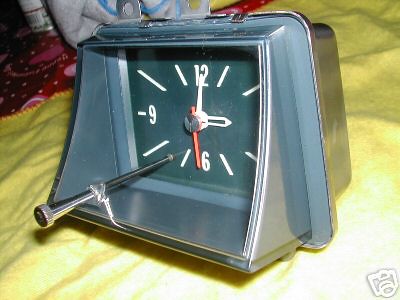This photograph captures a uniquely designed analog clock resting on a yellow blanket. The clock features a black and dark gray color scheme, with a striking blue front face. It has distinct white hour and minute hands, and a contrasting red second hand. The face of the clock prominently displays the numbers 12, 9, and 6, while lines mark the positions of the other hours. Notably, where the number 3 would be, a metallic rod appears to protrude through the clock face. The clock is mounted on a stand, suggesting it’s designed to sit on a desk. In the background, the scene is complemented by a red and pink fabric along with a gray sweatshirt, adding texture and depth to the setting. Additionally, a small white logo resembling a camera is visible in the bottom right corner of the image.